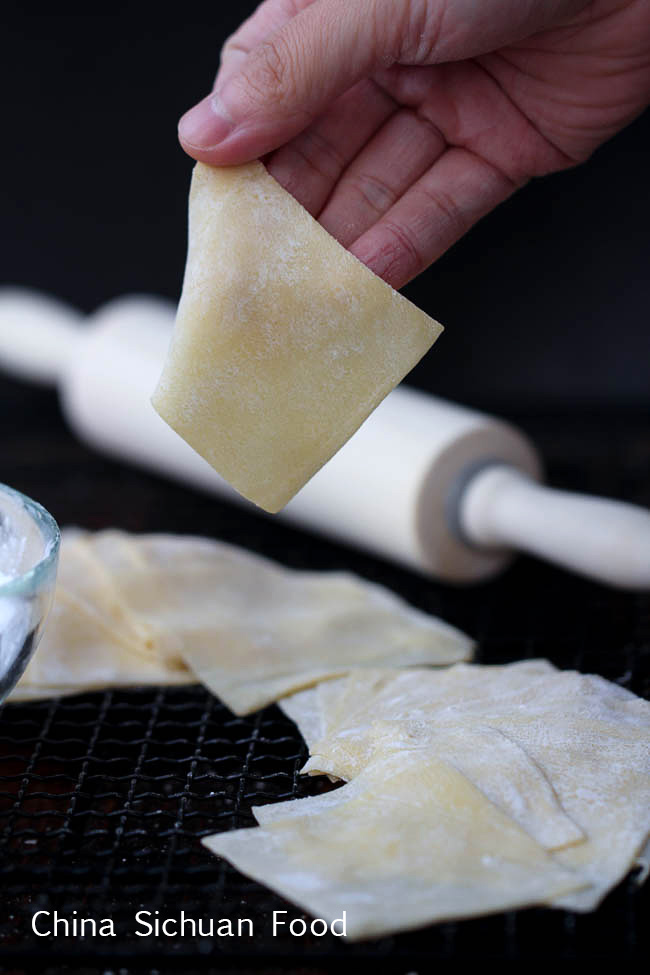The image is a detailed, rectangular photograph of someone in the process of making Sichuan cuisine. In the lower-left corner, white text reads "China Sichuan Food." The center of the image features a hand emerging from the upper right, holding a piece of square, yellowish pasta dusted with white flour to prevent sticking. Below this hand, several similar pasta squares are stacked on a black wire mesh, appearing ready for use. A wooden rolling pin, barely visible but essential to the pastry-making process, occupies the blurred background. Additionally, a partial view of a glass bowl filled with flour is visible in the left portion of the frame. The entire backdrop is dark, providing a stark contrast to the light-colored items in the scene, drawing attention to the meticulous preparation of what seem to be dumpling wrappers, integral to Sichuan culinary tradition.